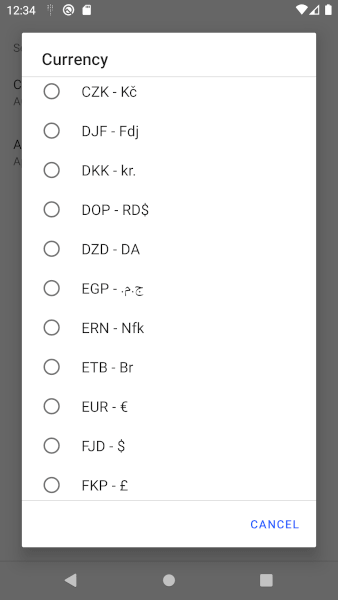This screenshot from an Android mobile device displays a pop-up selection menu overlaying a darkened background. The navigation bar at the bottom, identifiable by the standard Android navigation buttons—a triangle pointing left (Back), a circle (Home), and a square (Recent Apps)—confirms the device's Android operating system.

Prominently, the interface features a large white rectangular pop-up occupying most of the screen space, contrasting sharply with the dimmed background. At the top of this pop-up, bold black text reads "Currency," underscored by a thin gray line for emphasis.

Below this title, a sequential list of currency options is presented, each accompanied by a circular tickable selection button on the left. The listed currencies include CZK, DJF, DKK, DLP, DZD, and EGP, with additional unspecified currencies continuing the sequence. The user can choose their preferred currency by tapping one of these selection circles.

At the bottom of the pop-up menu, there is an option to dismiss the selection dialogue, marked by blue text reading "Cancel." This feature allows the user to exit the selection process without making any changes.